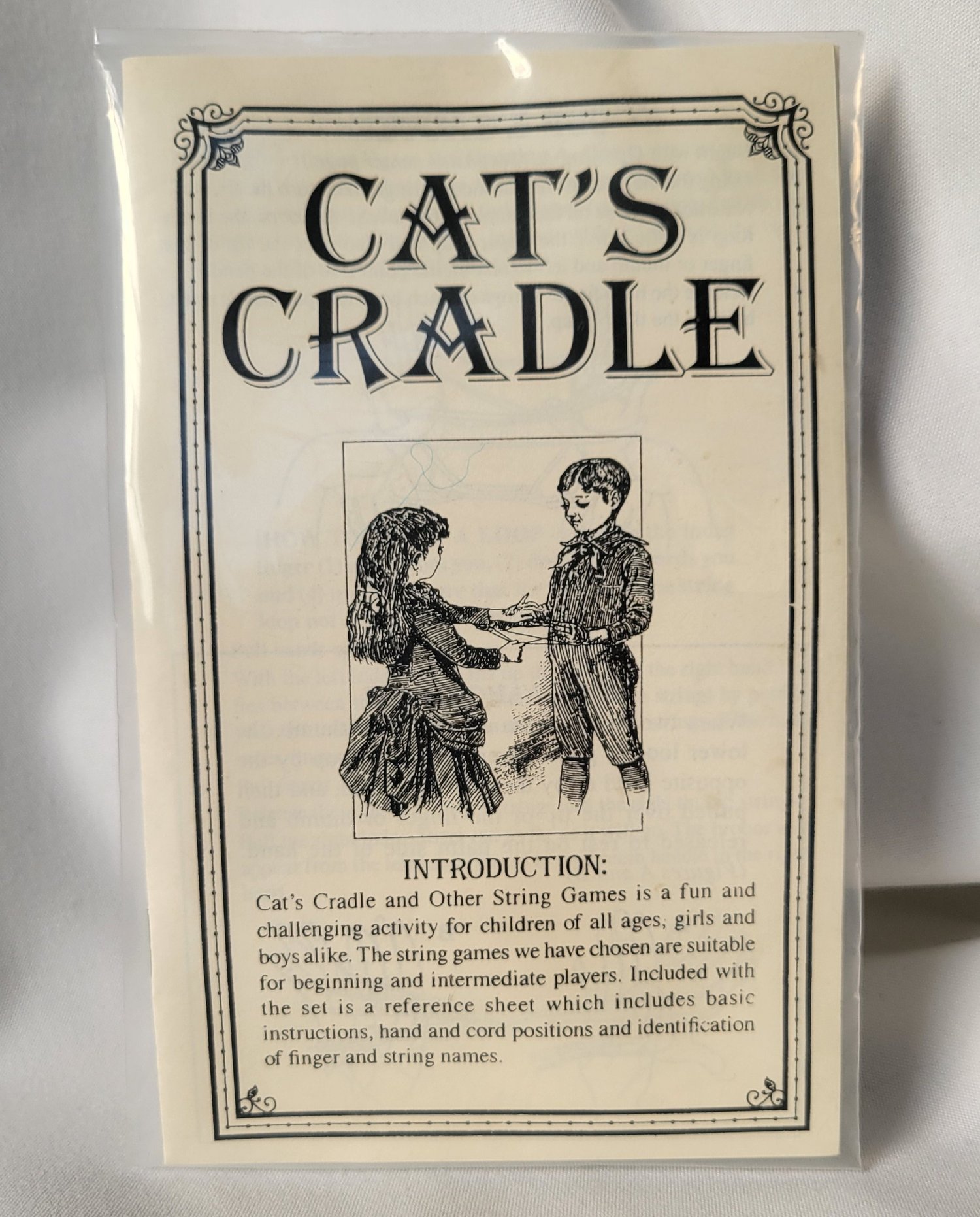The image is a color photograph of a brown paper-covered pamphlet encased in clear plastic wrap. The title "Cat's Cradle" is prominently displayed in black text at the top. Below the title, there is a detailed black-and-white illustration of a young boy and girl engaging in the Cat's Cradle string game. The boy, dressed in an 18th or 19th-century outfit with ruffled collared shirt, pants, and socks, stands opposite the girl, who has long hair tied with a ribbon and wears a dress with a ribbon sash at her waist. Their hands are intricately positioned with strings, indicating they are mid-game. Surrounding this central illustration is a decorative vine-like black line border. Below the illustration, the text reads:

"Introduction. Cat's Cradle and other string games is a fun and challenging activity for children of all ages, girls and boys alike. The string games we have chosen are suitable for beginning and intermediate players. Included with the set is a reference sheet which includes basic instructions, hand and cord positions, and identification of finger and string names."

This nostalgic composition subtly hints at the era through the children's clothing and adds a historical charm to the playful theme of the string games.